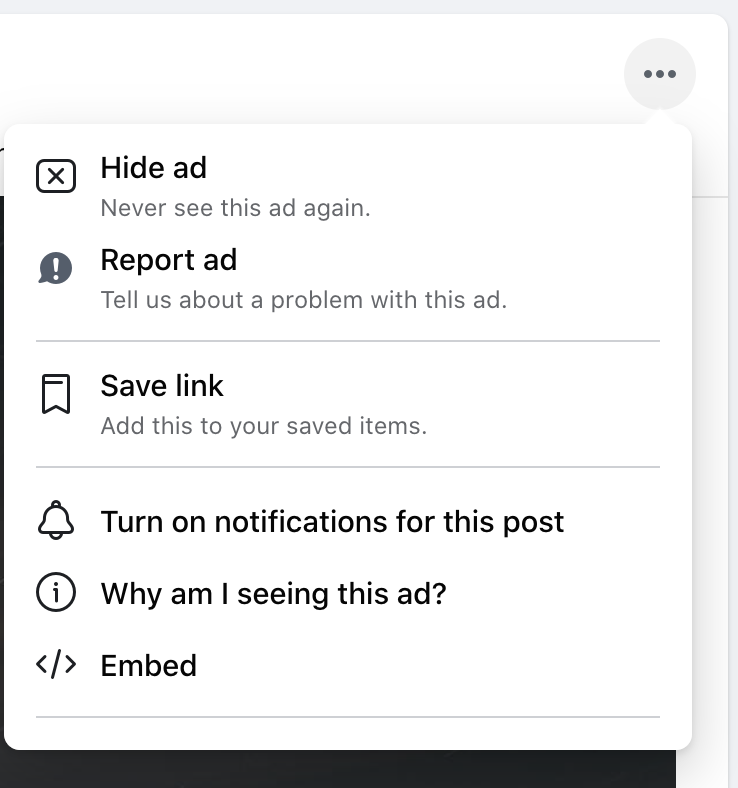This image is a cropped screenshot capturing the top-right corner of a webpage, specifically focusing on a pop-up menu originating from the menu icon. The pop-up menu contains several options for interacting with an advertisement. The options listed in the menu, each accompanied by a corresponding icon, include:

- "Hide ad" with an X icon
- "Report ad" with an exclamation point icon
- "Save link" with a bookmark icon
- "Turn on notifications for this post" with a bell icon
- "Why am I seeing this ad?" with an information icon (a circle with an eye)
- "Embed" with an icon featuring a left-pointing arrow, a forward slash, and a right-pointing arrow

The background of the original webpage is slightly visible as a black strip at the bottom of the screenshot, indicating that the image has been cropped.